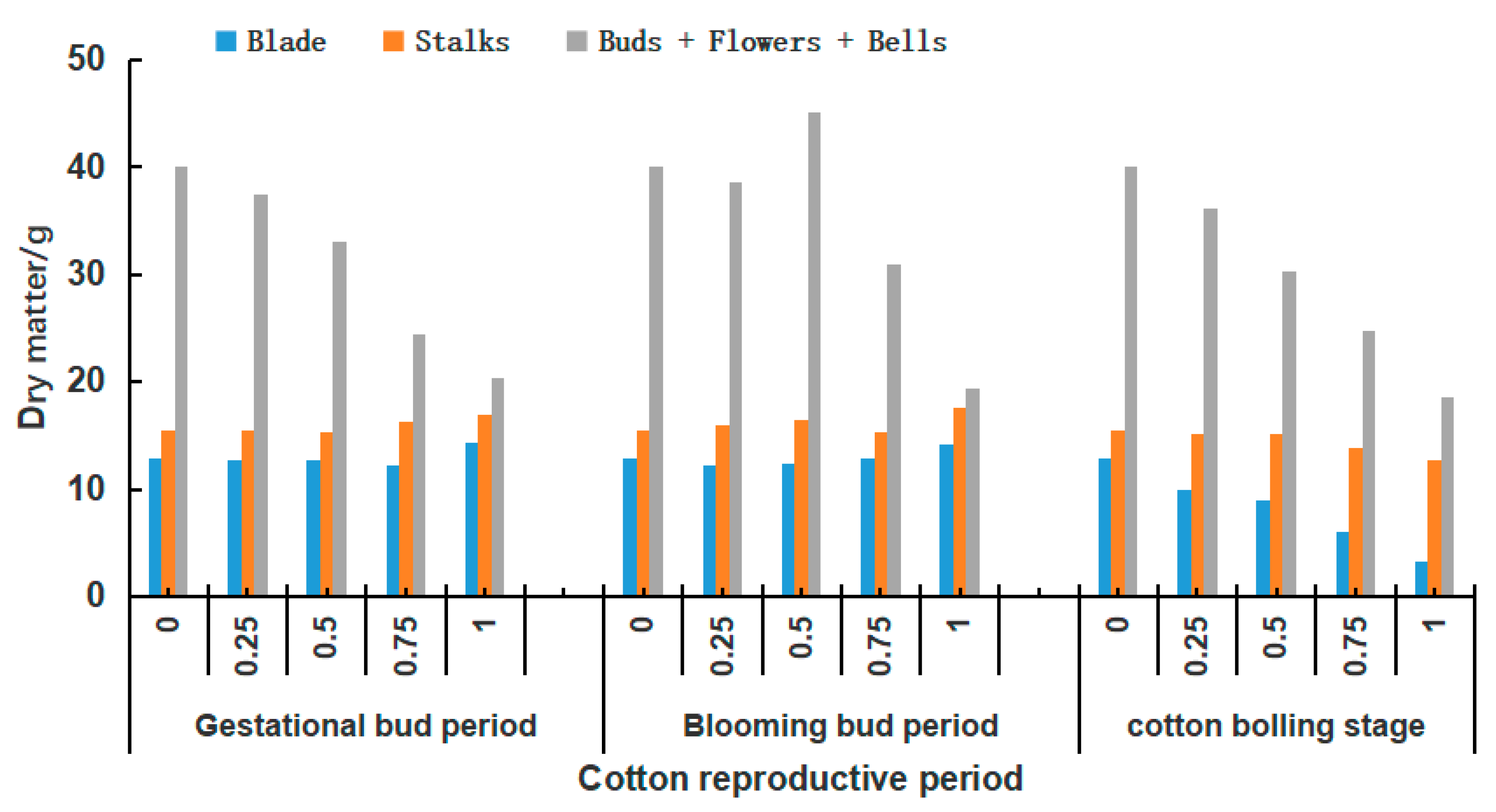The image displays a detailed bar chart focused on the cotton reproductive period, with "Dry Matter (grams)" labeled on the left side and an axis ranging from 0 to 50 in increments of 10. The chart is divided into three distinct sections along the bottom: gestational bud period, blooming bud period, and cotton boiling stage. This partition is marked at intervals of 0.25 from 0 to 1.

A legend at the top of the chart identifies three different colored bars: blue for blade, orange for stalks, and gray for buds, flowers, and bells. According to the chart, the gray bars, representing buds, flowers, and bells, show the highest dry matter content, followed by the orange bars for stalks, and the blue bars for blades, which have the smallest dry matter content. Overall, the chart provides a comprehensive visual analysis of the dry matter distribution among different components of cotton during its various reproductive stages, indicating the highest concentration in buds, flowers, and bells. The scientific nature of the chart suggests it could be from a science manual, medical manual, or an article discussing cotton reproduction.